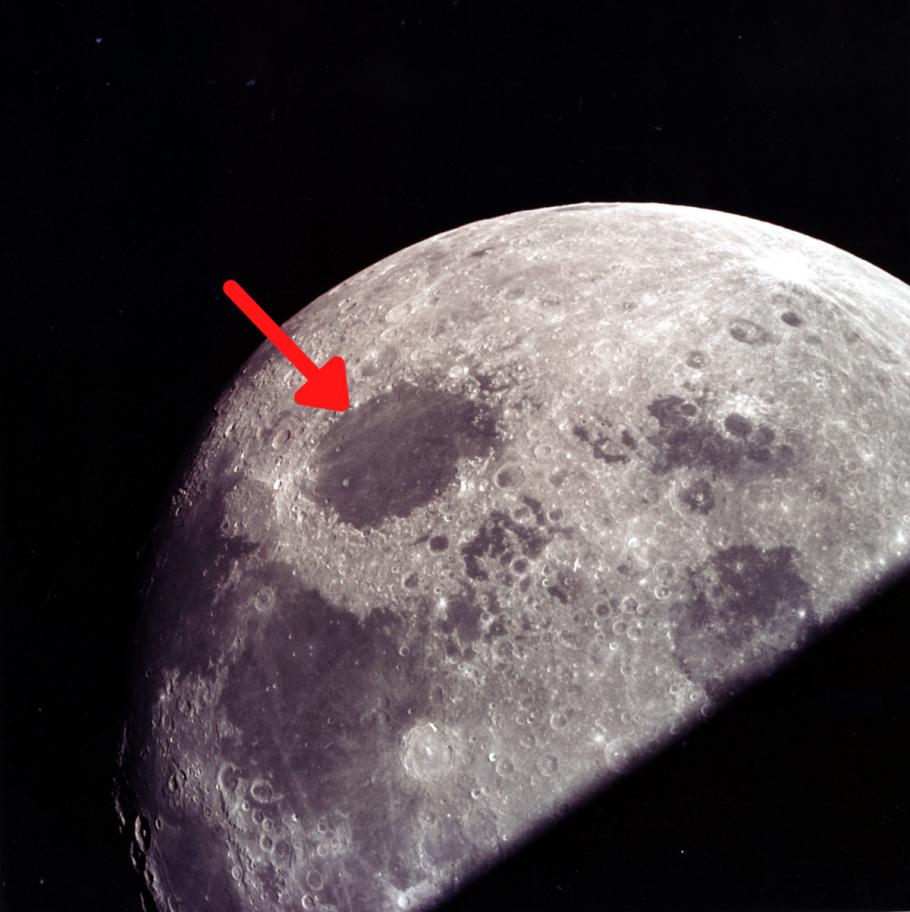This black-and-white photograph of the Moon presents a detailed close-up view, emphasizing the lunar surface's texture and crater formations. The Moon occupies most of the frame, slightly off-centered and leaning towards the right. The illuminated right side of the Moon contrasts sharply with the dark shadows along the lower left and bottom right, suggesting the dividing line between the lunar day and night, often referred to as the terminator. Craters of varying shades of gray decorate the surface, with a notable brighter, almost circular, white area near the top. The background is a stark black, dotted with the occasional star. A prominent feature of the image is a large gray mass near the top center, highlighted by a bright red arrow pointing at this specific area, though the reason for this emphasis is not explained. This image, marked by its detailed portrayal of the Moon's features and the vivid red arrow, suggests it could be used for educational or scientific purposes related to space exploration.